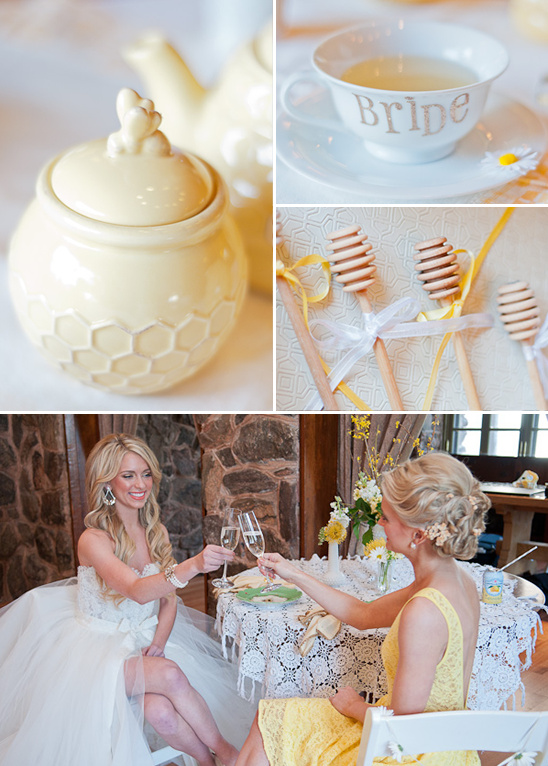This is a vertically oriented, wedding-themed photograph divided into four sections. In the top-left, there's a close-up of a cream-colored honeycomb-patterned jar with a beige tea kettle blurred in the background. The top-right section features a white teacup with gold lettering that reads 'Bride,' placed on a matching white saucer with a white daisy beside it. Below this image are four honey sticks, each tied with alternating white and yellow ribbons, laid out neatly on a white table. The bottom half of the image showcases two young adult women, both white with long blonde hair, sitting across from each other at a table with a white floral tablecloth. The bride, identifiable by her white dress and large earrings, holds a champagne flute mid-toast with the other woman, who is likely the maid of honor, wearing a yellow dress. A rock wall with an opening for windows can be seen in the background, suggesting this is likely a cozy and intimate bridal shower setting.